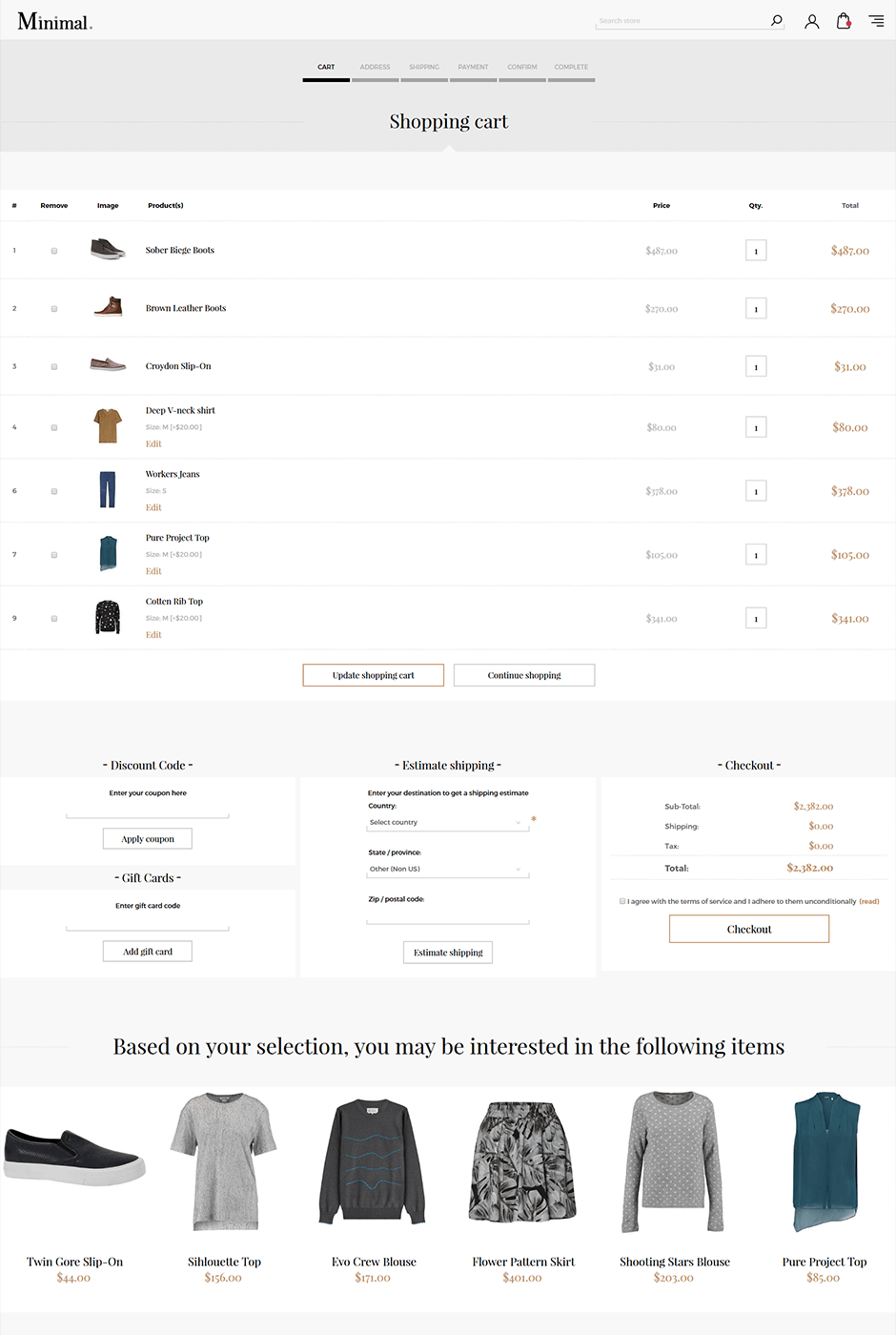This image is a screenshot likely taken from a computer, oriented in portrait mode and characterized by a vertical layout that's significantly taller than it is wide. The predominant colors in the screenshot are darker gray, light gray, and white. 

At the very top, a lighter gray horizontal border spans across the image. Within this border, the word "minimal" is displayed in black text on the left-hand side. Adjacent to it, towards the right, there is a search bar, followed by icons that include a person icon, a shopping bag icon with a red notification dot, and a hamburger menu icon sequentially aligned.

Beneath this top border, the word "different" is displayed, possibly indicating a section or heading. Below this, there is a darker gray elongated box containing various categories. These categories are largely grayed out and illegible, except for the first category which is slightly clearer but still not distinctly readable.

Further down, the text "shopping cart" is prominently displayed in black, below which lies a gray horizontal border devoid of any content. Beneath this border is a white box-like area divided into multiple columns. The columns are labeled as follows: 
1. A pound sign (#) indicating the item number, listed from one to nine.
2. "Remove" with adjacent checkboxes for removing items.
3. "Image," displaying the images of the clothing items purchased.
4. A column starting with the letter 'P,' though the complete word is not discernible.
5. "Price," detailing the cost per item.
6. "Quantity," showing the number of each item.
7. "Total," reflecting the total cost multiplied by the quantity.

Below these columns, there are options such as "Update Shopping Cart" and something pertaining to shipping, followed by a "Checkout" button. At the very bottom, the total cost of the shopping cart is displayed.